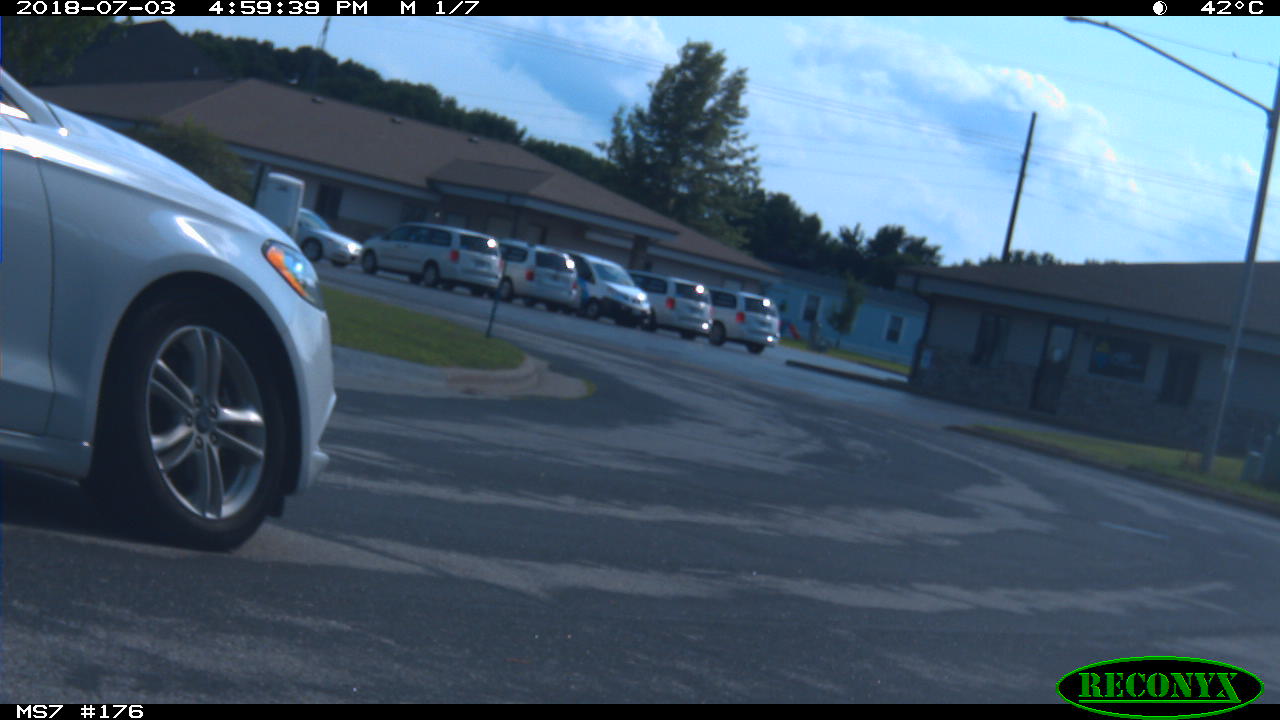The photo depicts a daytime scene on a road situated near two light brown business buildings, with a light blue house visible in the distance. A partly visible silver car is entering the frame from the left, and a line of parked vehicles, including minivans and SUVs, is positioned in front of one of the business buildings. The image shows a small grassy area near the road's curb, and various street lights and power lines are visible. The sky is slightly clouded, with indications that it may be nearing dusk. There is a timestamp in the upper left corner reading "2018 703 at 4:59 p.m." along with a temperature indication of 42 degrees Celsius. In the bottom right corner, a black oval logo with green lettering spells out "Reconyx." The bottom left side of the image contains the text "MS7176."